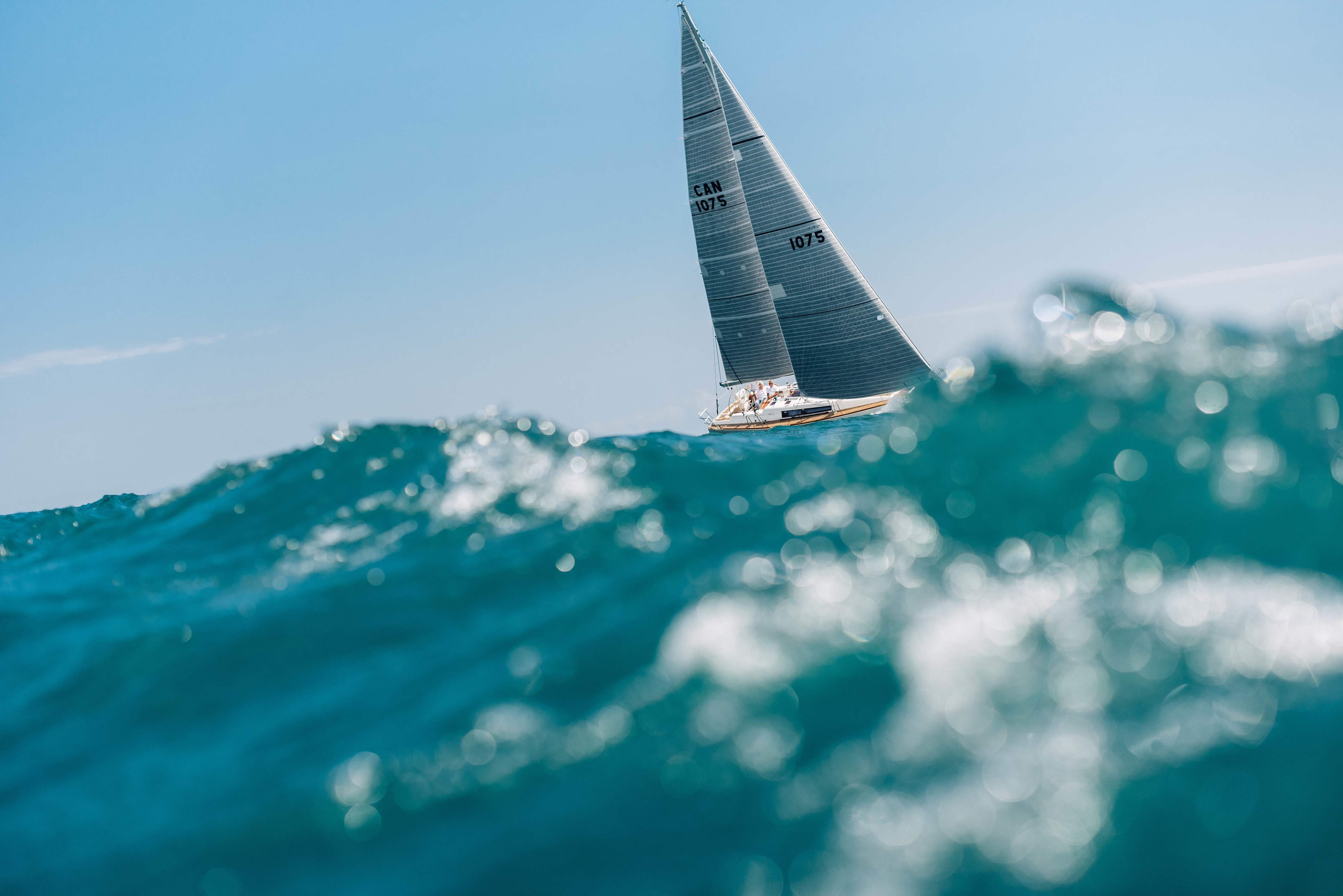This photograph captures a dynamic scene of a sailboat out at sea on a bright, sunny day. The image has a unique perspective, as if the camera is partially submerged, rendering the water in the immediate foreground blurry due to proximity. The sailboat, which is slightly off-center to the right and leaning towards the camera, is sharply in focus. It appears to be under the influence of a strong wind, creating an impression of movement and energy. The boat is white with two large sails; the left sail bears the inscription "CAN 1075" and the right sail simply "1075." The sky above is a serene blue with light, wispy clouds enhancing the sense of openness and freedom. Three small figures are visible on the boat, presumably wearing white, though they are not easily discernible due to their size in the composition. The photograph contrasts the smooth, clear, blue ocean with pockets of white foam, suggesting the boat is navigating actively through the water, creating a vibrant and engaging maritime scene.